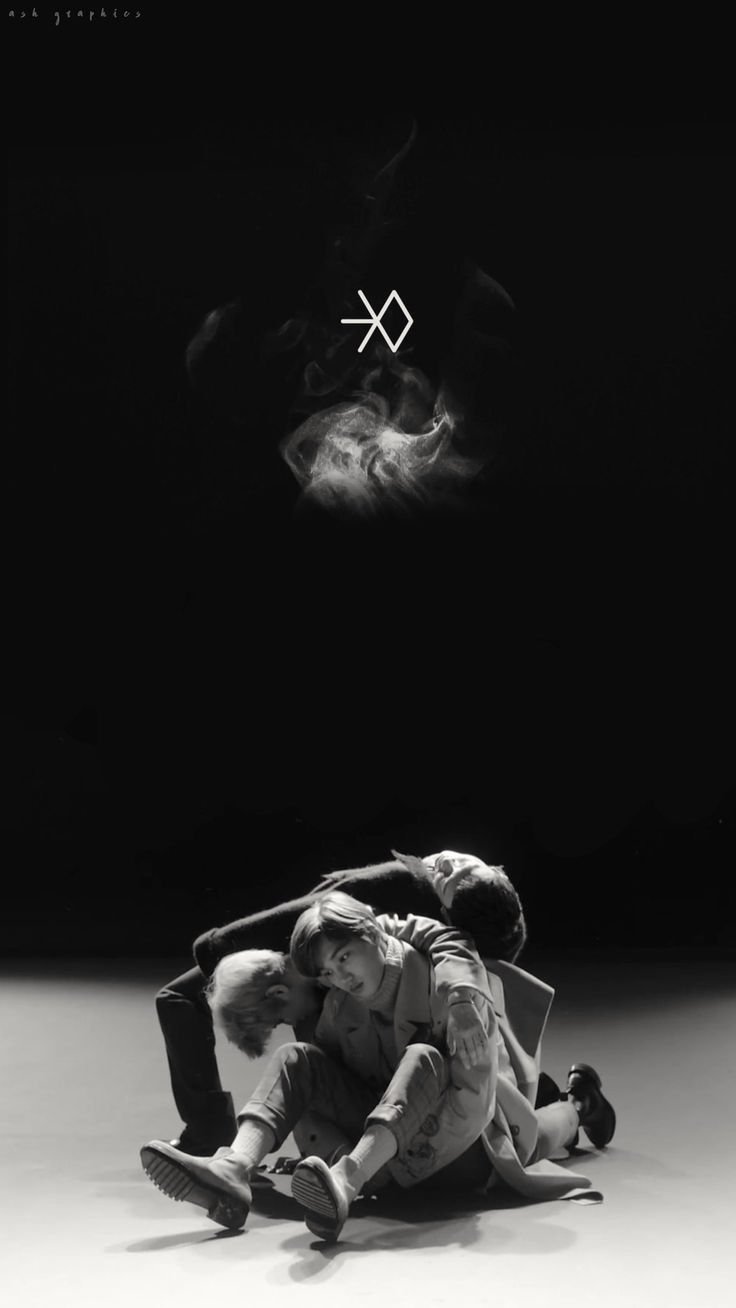In this detailed black-and-white photograph, three young adult members of a K-pop group, likely EXO, are intertwined in a complex pile on the ground. The main subject, possibly Kai, sits with his legs outstretched, head bowed close to his knees, and arms wrapped around his legs. He is wearing a gray shirt and is barefoot. Another individual is draped across him, their chest pressed down and arms encircling his legs. Above them, a third person lies on their back, with dark brown hair and wearing a black suit. The background transitions smoothly from light gray at the bottom to black at the top. At the top center, a white puff of smoke hovers, above which is the group's logo—a diamond shape with three white lines extending from the left side, one pointing up, one down, and one straight to the left. The evocative and artistic composition, with its somber and surreal atmosphere, encapsulates the unique aesthetic of the group.